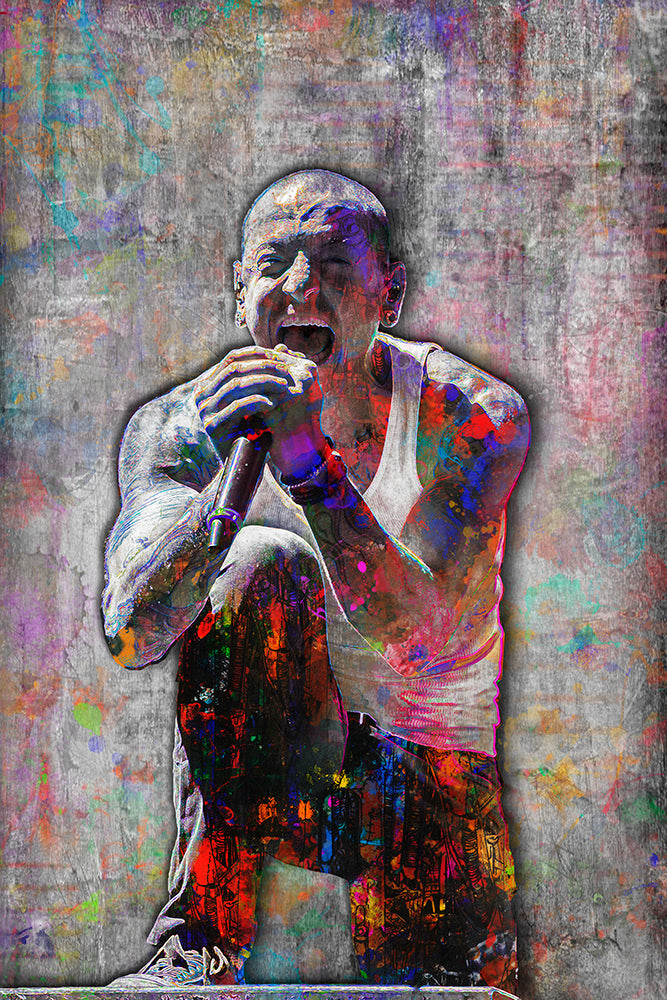The image is a vibrant, abstract artwork of Chester Bennington, the lead singer of Linkin Park. It's a photorealistic portrayal with splashes of vivid colors. The background is textured gray, enhancing the dynamic paint blotches in shades of blue, pink, red, orange, green, yellow, and purple that streak across the image. Bennington, with a shaved head and large round earrings, is captured in an electrifying moment, his mouth wide open and eyes almost closed, passionately screaming into a microphone held tightly in both hands. He wears a white sleeveless tank top, revealing tattoos on his arms, dark-colored pants with hints of red, gold, and blue, and white sneakers with distinct white laces. One foot is propped up on a stand. The chaotic yet intentional splatters of color vividly contrast with the photorealistic depiction, giving the artwork a surreal, cartoonish feel.